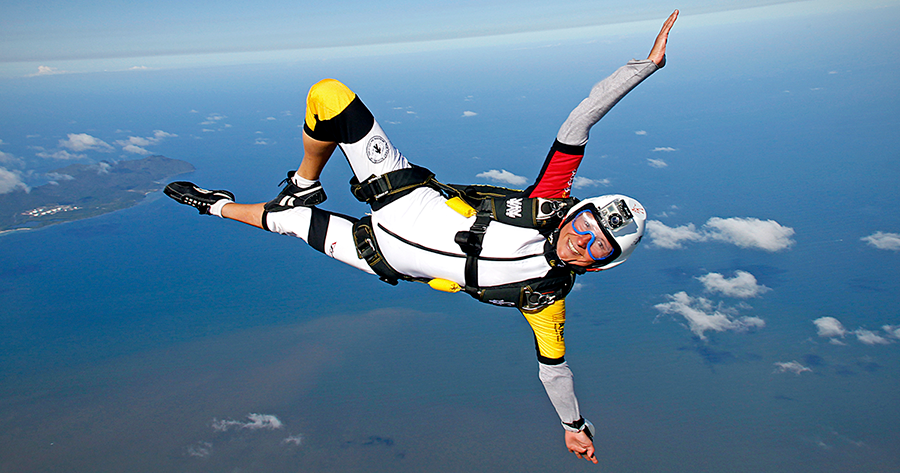The image captures a skydiver mid-fall, suspended in the air before deploying their parachute. The person is posing horizontally, with arms stretched outward in a T-position and one leg bent upwards. They are dressed in a white suit featuring distinctive black straps, a black front zipper, a yellow armband on one sleeve, and a red armband on the other. Their gear includes a black parachute harness, a white helmet, clear goggles, and black shoes. The scene is set against a backdrop of a clear blue sky with scattered fluffy white clouds below. Some grayed-out land is visible in the distance, adding depth to this exhilarating moment captured either by another skydiver or from an airplane. The skydiver’s outfit and midair pose convey a sense of excitement and adventure.